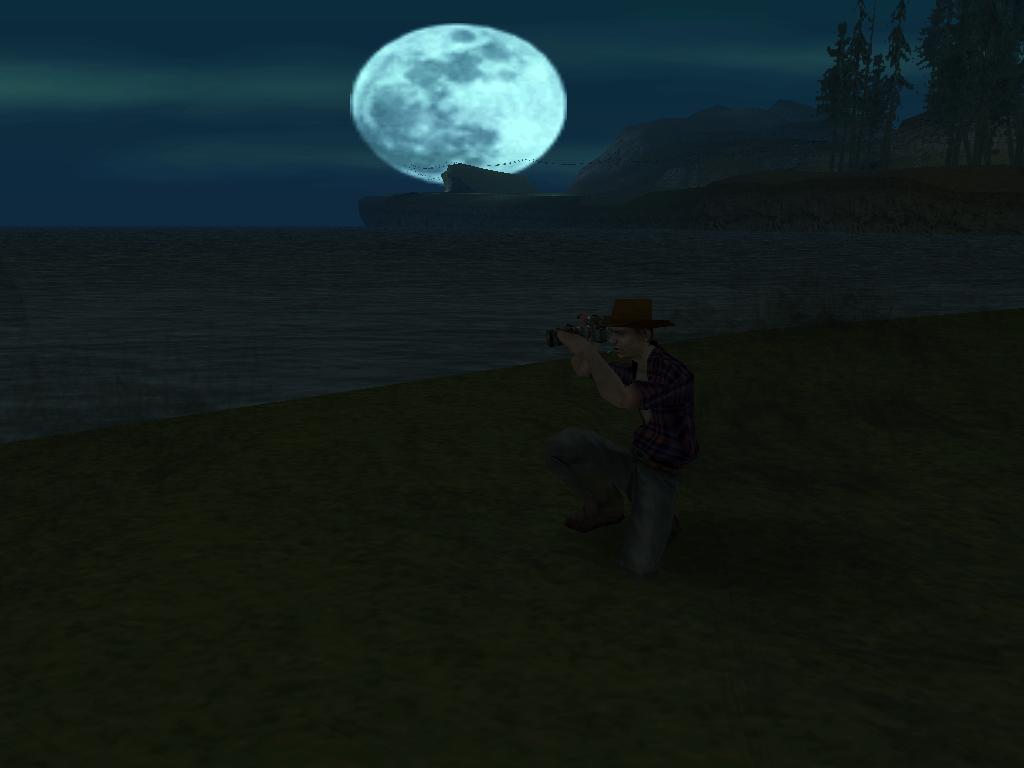In this digital or video game-inspired scene, a character is depicted kneeling on a grass-covered terrain. They are adorned in a classic cowboy hat, a plaid shirt, and jeans, conveying a rugged, outdoorsy appearance. The individual is poised to capture a moment through a camera, aiming it towards the surrounding scenery. Behind them stretches a serene body of water, its surface reflecting the subdued light from the environment. Across the water lies a tranquil shoreline, adorned with rolling hills and scattered trees that add to the scenic beauty. Dominating the background is an enormous, luminous moon, casting a radiant glow amidst a dark, cloudy sky. The interplay of light and shadow in this nocturnal setting creates a captivating and mystical atmosphere.